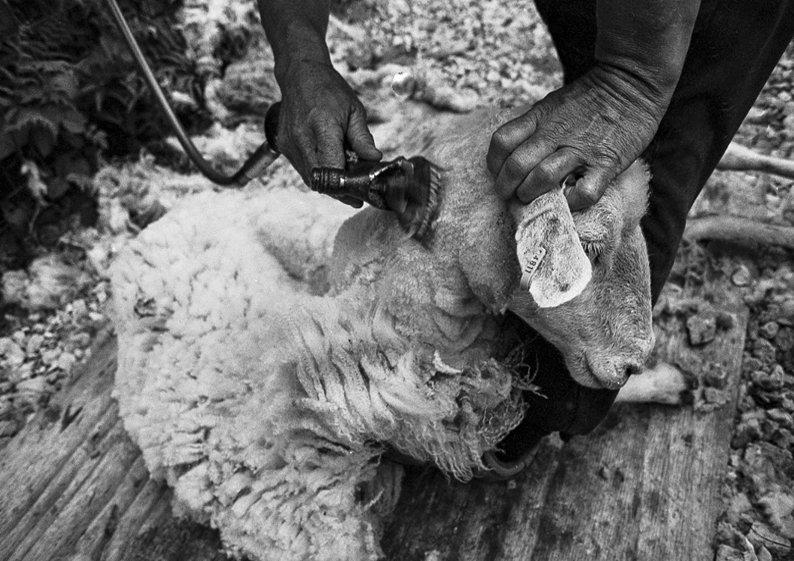This vintage black and white photograph, possibly taken outdoors, captures an intimate moment of sheep shearing. A white lamb, lying on a wooden platform amidst a gravel ground, is being held and sheared by a dark-skinned man. The man's left hand firmly grasps the top of the lamb's head while his right hand maneuvers an electric shear, buzzing with an older style, to remove the wool. The lamb's fluffy body contrasts with its freshly shorn neck and head, indicating the precision and progress of the shearing. Scattered around are tufts of wool already removed, with the sheep's back legs and one front leg visible in the shot. The man’s attire includes dark, long pants, and though his shoes are barely visible, they appear to be running shoes. The photograph’s composition is focused on the lamb with the man's hands and parts of his legs entering from the edges, against a background of gravel and a faint bush in the upper left corner, emphasizing the shearer’s concentrated effort amidst a simple, rustic setting.